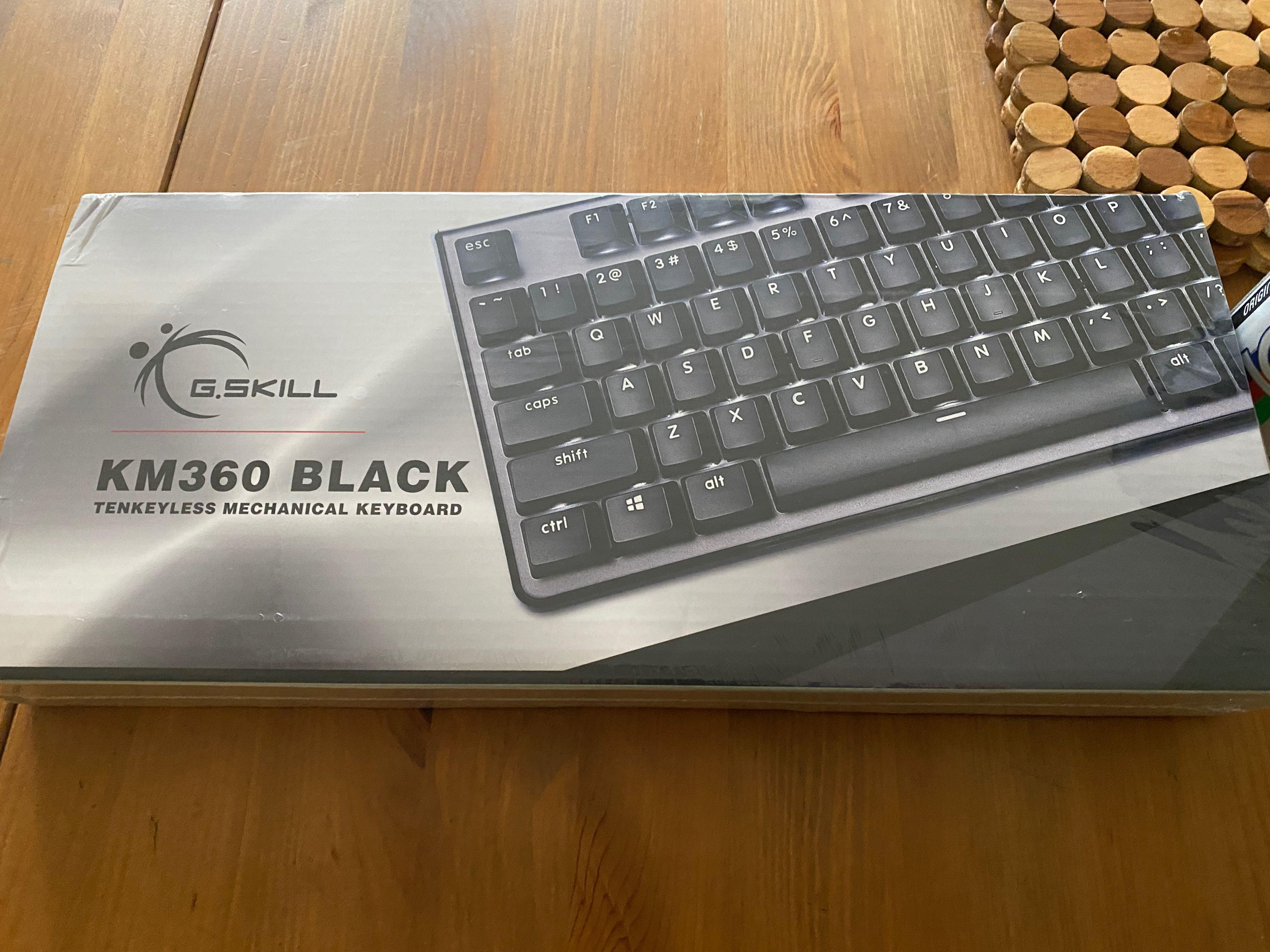On a horizontally aligned dark brown table with visible wood grain and varying shades of brown, there's a central focus on a slightly beat-up box. The box is gray at the top left, gradually transitioning to black towards the bottom right. In the upper right corner of the image, there is a black mechanical keyboard with white key lettering and a gray background. The keyboard is identified on its left side with the inscriptions "G. Skill" and "KM 360 Black 10-Keyless Mechanical Keyboard." Additionally, in the upper right part of the table, there appear to be stacked objects resembling wine corks made of different wood shades: light tan, darker tan, very light brown, and dark brown.